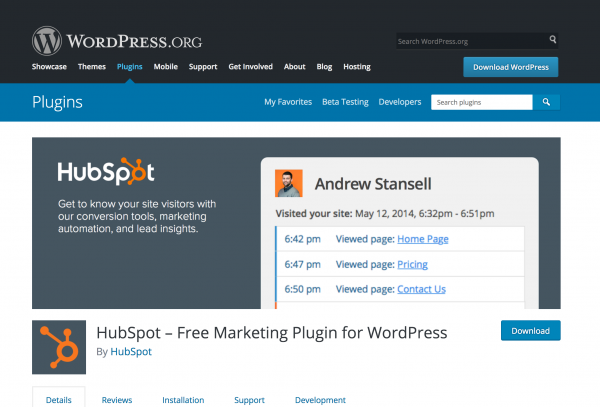This image captures a webpage from WordPress.org. The top of the page features a prominent black header with the WordPress logo ("W" emblem) and the text "wordpress.org." Alongside the logo, the menu options displayed in smaller print include: Showcase, Themes, Plugins, Mobile, Support, Get Involved, About, Blog, and Hosting. The "Plugins" menu item is highlighted, indicating it has been selected, revealing a blue submenu. The submenu options are My Favorites, Beta Testing, Developers, and a search bar labeled "Search Plugins." 

Above the black header is a notable blue "Download WordPress" button. Further down, a white line separates this section from a gray box. Inside the gray box, it introduces HubSpot with the text: "Get to know your site visitors with our conversation tools, marketing automation, and lead insights." A section within the gray box features an image of a man labeled Andrew Stenel, along with some informational content. There is also a download button included in this section.